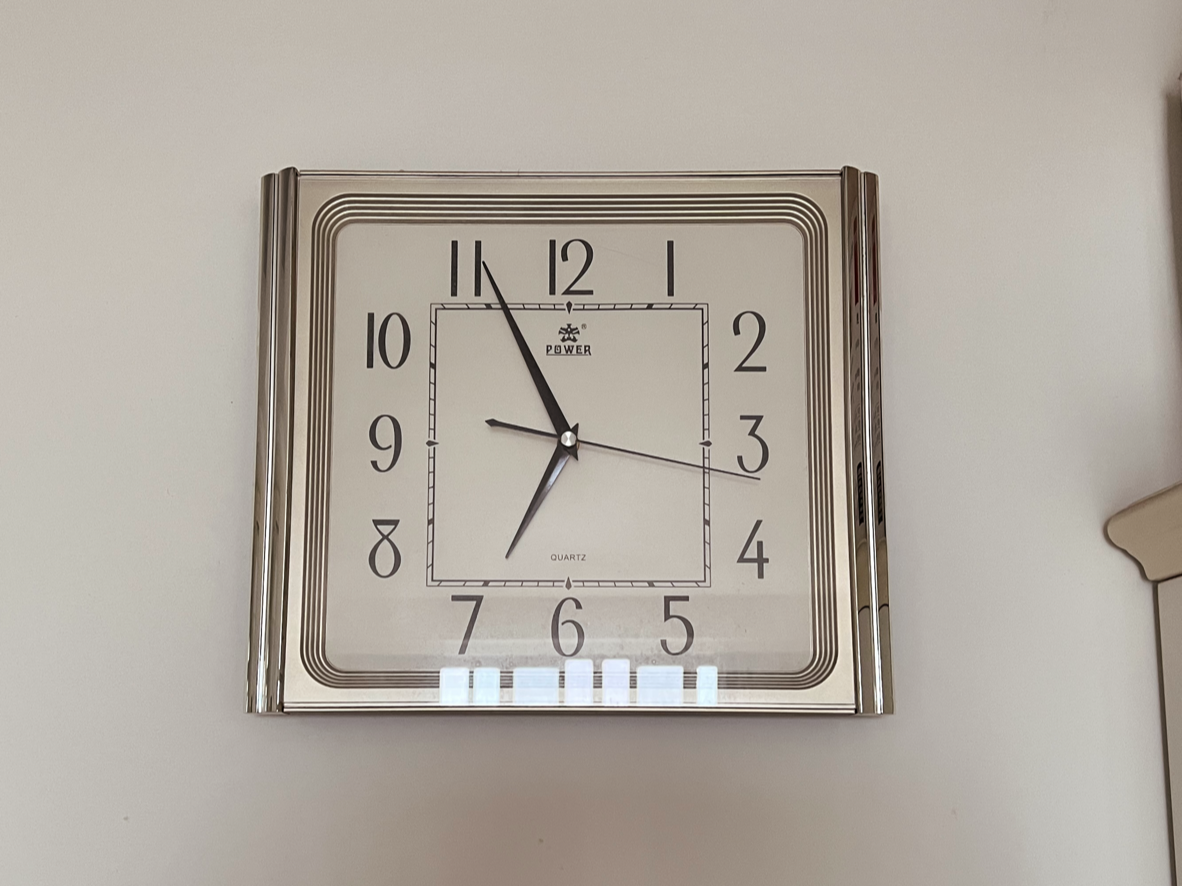A photograph features an elegantly designed clock, mounted flat on a wall. The clock, with its pewter-like silver frame encasing clear glass, reflects multiple windows behind it, adding depth and light to the scene. The clock's unique square shape distinguishes it from traditional circular clocks. All the numbers are legible and aligned upright, set against an off-white background. A sweeping second hand traverses the dial. To the right of the clock, the corner of what seems to be a mantel or possibly a picture shelf juts out, adding context to the interior setting and enhancing the overall composition.